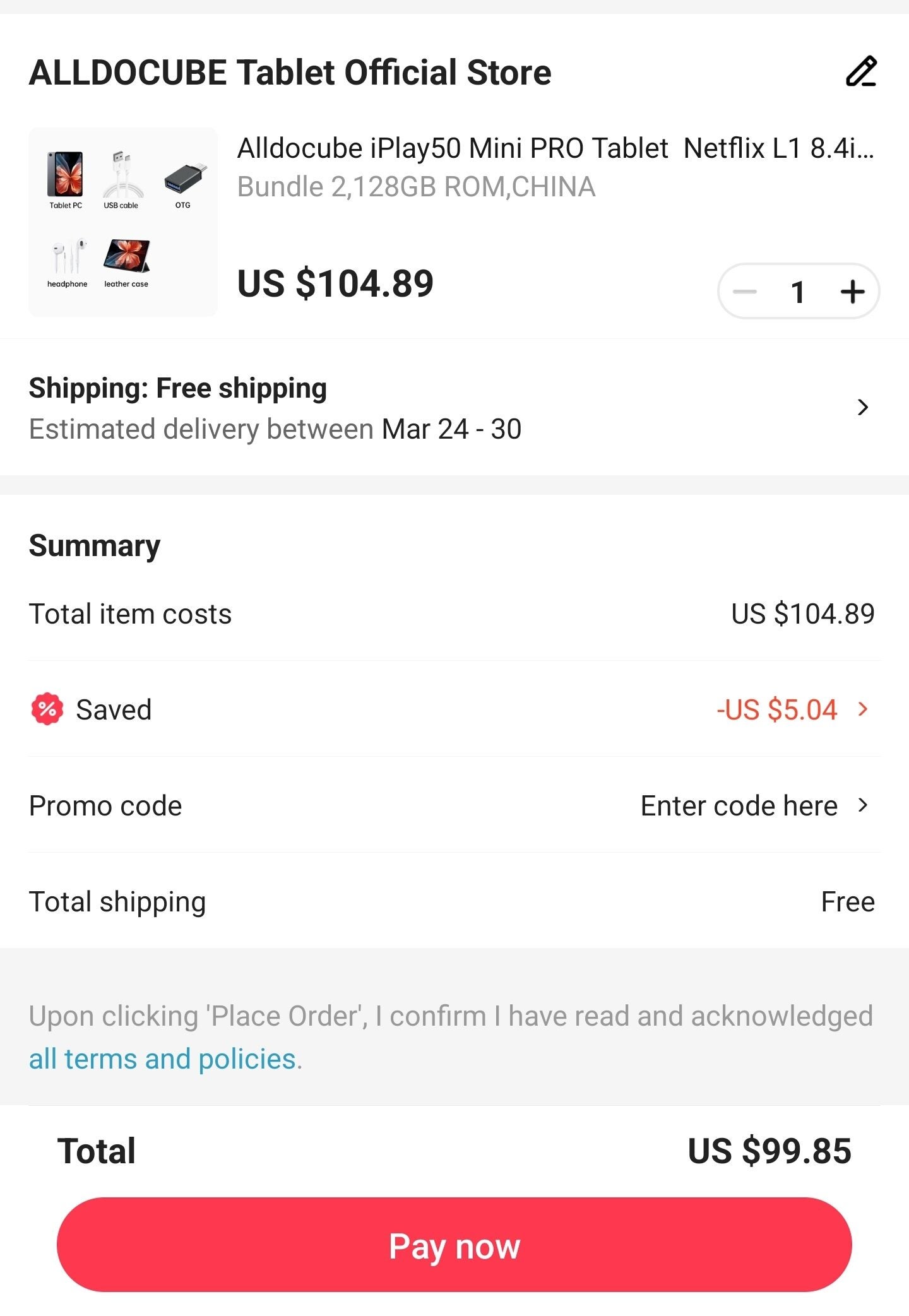A detailed screenshot showcases an online listing from the "All Do Cube Tablet Official Store". In the top left corner, black bold text states the store's name. Directly below, the "All Do Cube iPlay 50 Mini Pro Tablet" is highlighted, featuring specifications such as Netflix L1 compatibility, an 8.4-inch screen, and a storage capacity bundle of 128 GB, originating from China. The tablet is priced at US $104.89. A quantity selector button is visible on the right.

Further down, bold text announces "Shipping," confirming free shipping with an estimated delivery timeframe between March 24th and March 30th. A summary section breaks down the costs, listing the total items’ cost as US $104.89. An additional line with the word "Saved" and a percentage icon shows a discount of negative US $5.04. There is a field for entering a promo code. The total shipping cost is stated as free, bringing the overall total to US $99.85.